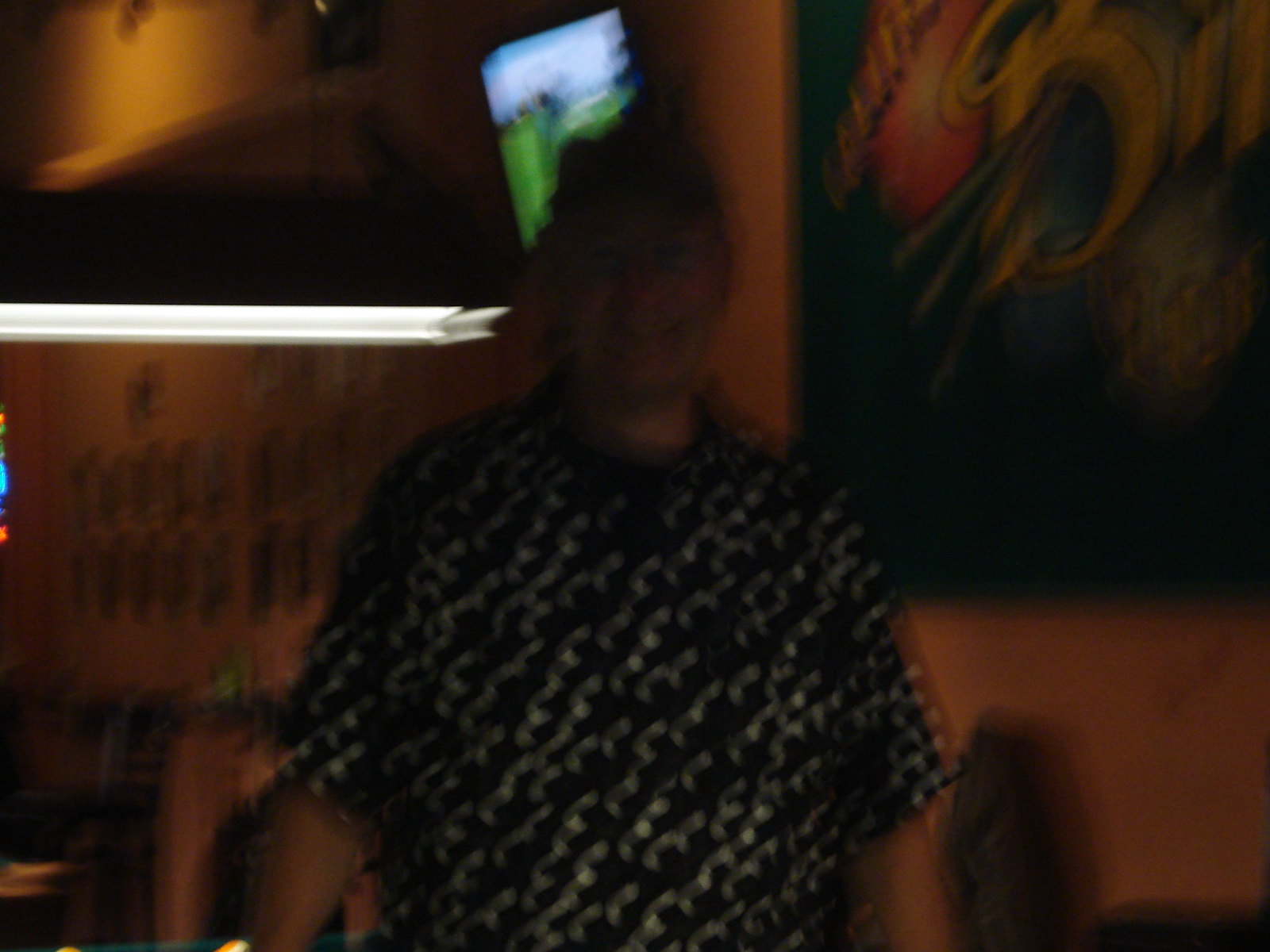This photograph, although blurred, captures a smiling man dressed in a short-sleeved black shirt adorned with white graphics. Above him, a dark-colored pendant light casts a soft, white glow. Behind his head, a television screen displays a mix of green, blue, and white colors. To his side, a decorative item with a green background showcases vibrant shades of light green, yellow, red, and blue. The background features additional blurred images, including photos mounted on the wall and indistinct black shapes, adding depth to the scene despite the heavy blur.